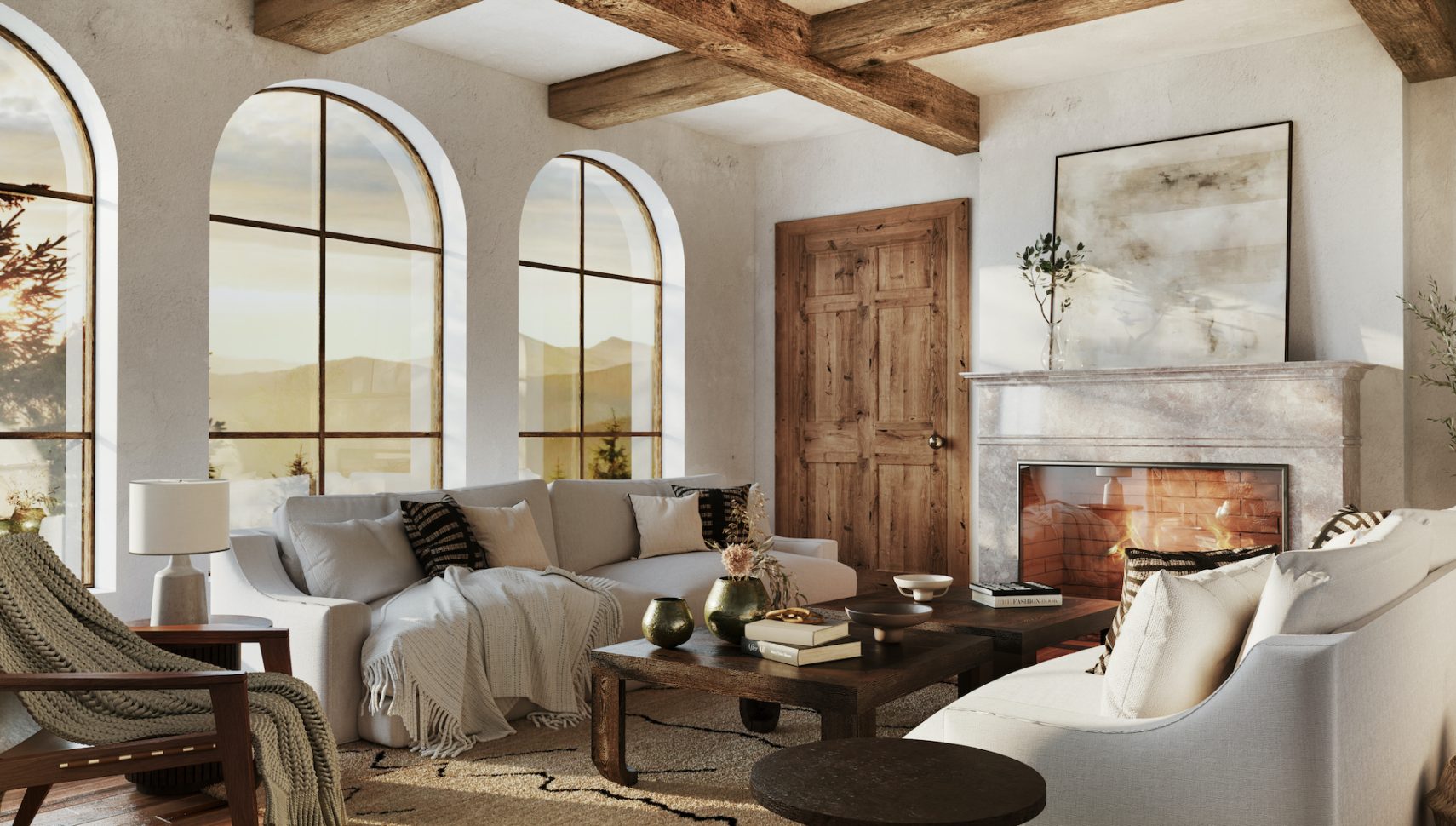The photo depicts a rectangular living room with a predominantly white color scheme highlighted by warm brown accents. The white walls and ceiling, which features exposed wooden beams, create an airy atmosphere. On the left wall, three rectangular arched windows offer a stunning view of a sunset over a mountain range. The room is furnished with two parallel white couches, adorned with a mix of white and striped black-and-yellow pillows. Between the couches are two brown square coffee tables. A marble fireplace, topped with a blank square mural, sits between the couches, adding elegance to the space. A wooden chair with a blanket draped over it is positioned to the left, while a side table with a lamp stands to the right. Additionally, a large wooden door is located off to the right behind the second couch. The room blends its crisp white palette with natural brown touches, providing a cozy yet sophisticated ambiance.